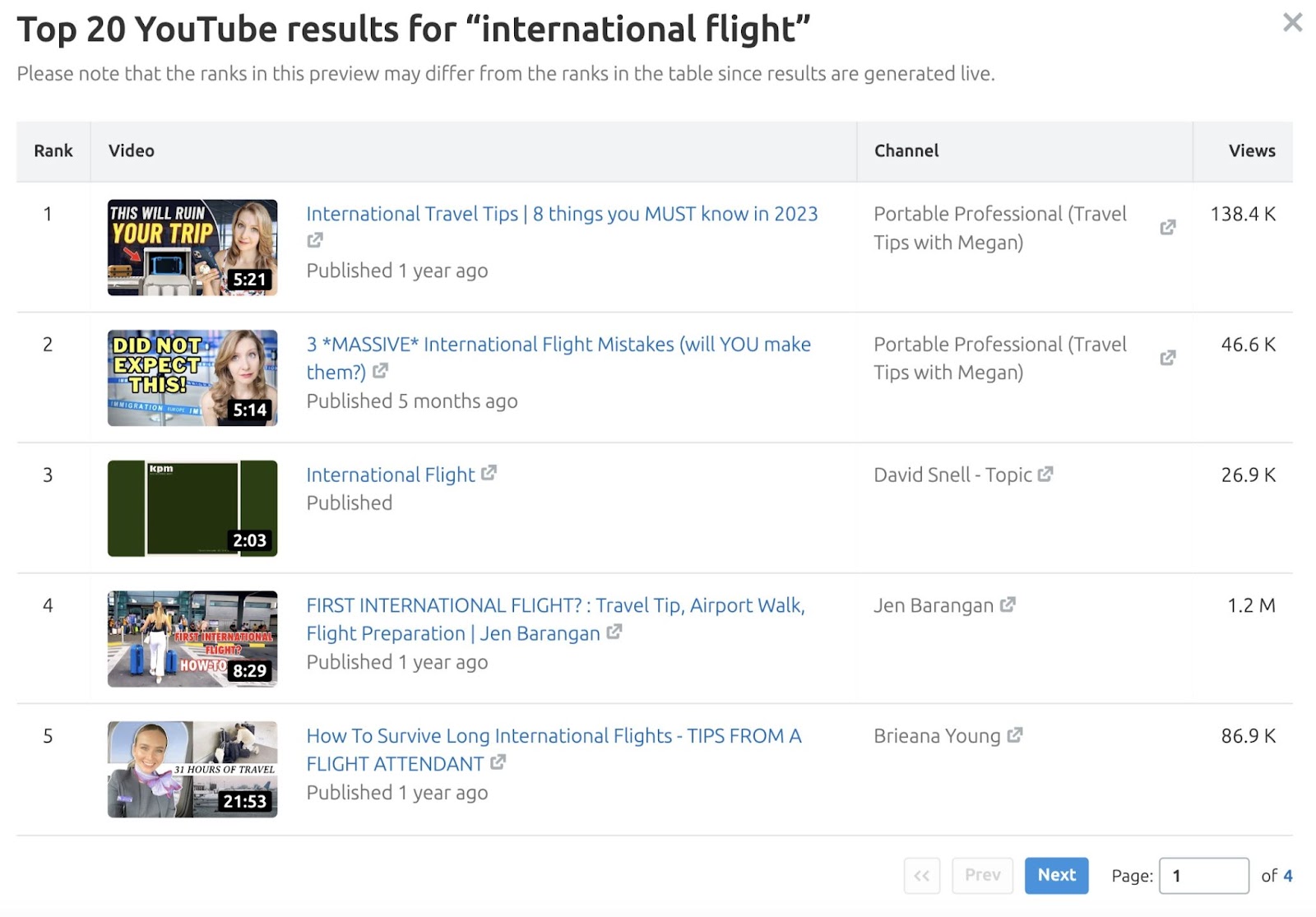Here are the search results for international flight tips. At the top, it says, "Top 20 YouTube results for an international flight," and below that, a note informs users that the ranks in this preview may differ from those in the final list since results are generated live.

The headers of the table, displayed in black text, read: Rank, Video, Channel, and Views. The search results, ranked 1 through 5, are displayed with screenshots of the respective videos on the left and related information on the right, linked in blue text.

1. **International Travel Tips: 8 Things You Must Know in 2023**
   **Channel:** Portable Travel Tips with Megan
   **Views:** 138,000
   Thumbnail: A woman making an intrigued face with the text "This Will Ruin Your Trip."

2. **I Did Not Expect This: Lines at the Airport**
   **Channel:** Portable Professional Travel Tips with Megan
   **Views:** 46,000
   Thumbnail: The same woman with the text "I Did Not Expect This."

3. **Massive International Flight Mistakes: Will You Make Them?**
   **Channel:** David Snell
   **Views:** 26,000
   Thumbnail: A view of the airport with people lined up.

4. **First International Flight? Travel Tips, Airport Walk, Flight Preparation**
   **Channel:** Jen Berengan
   **Views:** 1.2 million
   Thumbnail: A woman walking across a street with a green screen background.

5. **How to Survive Long International Flights: Tips from a Flight Attendant**
   **Channel:** Brianna Young
   **Views:** 86,000
   Thumbnail: A flight attendant offering advice.
   
At the bottom of the table, there's a "Next" button for more results. The current page being viewed is page 104.